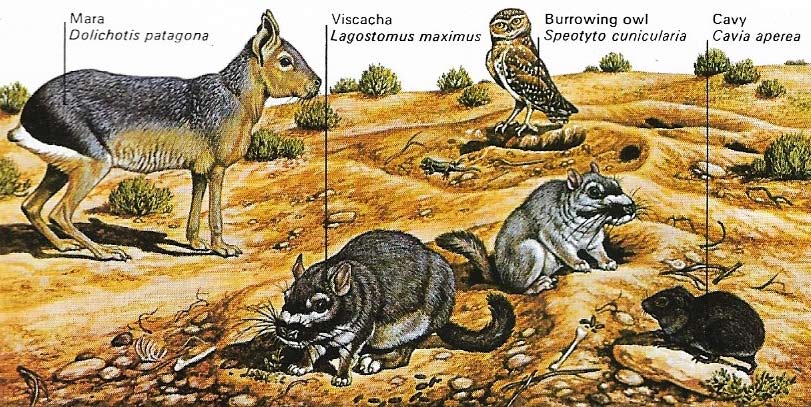In this detailed illustration, rendered with pen and ink alongside watercolor or gouache, five distinct animals are labeled within a barren desert setting adorned with sparse puffs of greenery and sagebrush. The illustration, potentially for a textbook or nature biology book, presents each animal with thin, solid black lines connecting them to their identifying text.

In the foreground to the left, a brown Mara (Dolichotis patagonum) with black hair atop its head, pointy ears, and a flat nose faces right, showing its right profile. Moving rightward, another foreground creature is a black Vizcacha (Lagostomus maximus) with a white stripe across its face and a curled tail, slightly turned left but facing forward. Further right, and more forward, is a small black Cavy (Cavia aperea), facing left and showing its left profile.

In the background, a Burrowing Owl (Speotyto cunicularia), oriented toward the viewer but slightly turned to display its left side, adds to the detailed depiction of this arid environment. Bones scattered in the foreground contribute to the aged and desolate feel of this scientific illustration.